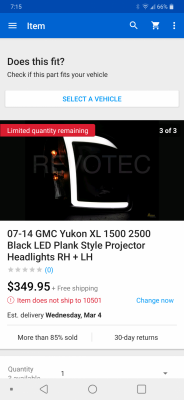This screenshot from a website depicts a detailed product listing page. At the top, a dark blue banner does display indicators, including the date (7-15), a Bluetooth symbol, battery life at 66%, cell signal strength, and a Wi-Fi signal. Immediately below, a slightly lighter and thicker banner features the label "item," a menu icon comprising three horizontal lines stacked vertically, a magnifying glass symbol for search, a shopping cart icon, and a vertical ellipsis.

The main content starts with a light gray background featuring the question "Does this fit?" in black text, directing users to check if the part fits their vehicle. Below this, a white banner with blue text in capital letters instructs users to "SELECT A VEHICLE."

The lower section shows a black background stating "3 of 3" and contains a red banner with white text indicating a "Limited quantity remaining." The product details are highlighted, with "REVOTEC" specified on the black background and the description "07-14 GMC Yukon XL 1500/2500 Black LED Plink Style Projector Headlights RH + LH" following. The item is listed at $349.95, with free shipping noted underneath.

Additionally, a disclaimer in red text informs that items are not shipped to the zip code 10501. Finally, the estimated delivery date is provided as "Wednesday, March 4th," with an option to "change now" in blue text beside it.